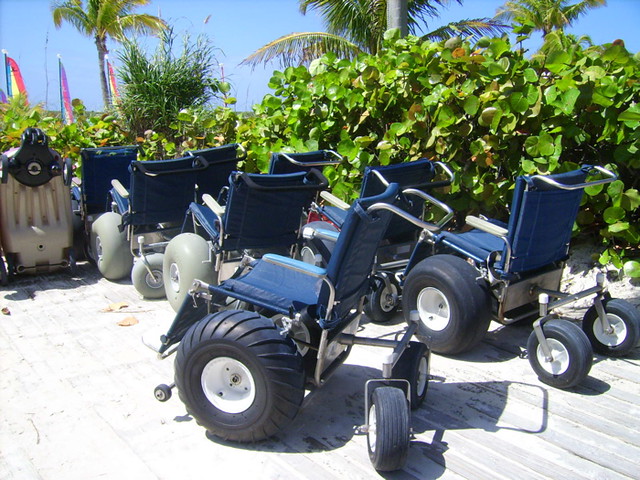The image is a color photograph taken near the beach, as evidenced by the tall parasails and palm trees visible in the background. The foreground showcases an array of uniquely designed wheelchairs lined up on a wooden deck. These wheelchairs feature navy blue seats and backrests, emphasizing their comfort and durability. Unlike traditional wheelchairs with metal spoked wheels, these are equipped with large, rubberized wheels with deep treads, similar to those found on water buggies, making them suitable for navigating sandy beaches. Additional design elements include smaller, supportive rear wheels and very small front wheels positioned at a 45-degree angle to prevent tipping. The wheelchairs also have stainless steel rounded poles at the top for easy pushing or pulling. The wooden deck underneath them is a light grayish-white pine, partially obscured by sand or appearing very pale due to overexposure on the left side of the image. In total, there are roughly ten to eleven wheelchairs, with a few of them featuring smoother gray wheels. The tropical setting, with its lush foliage, palm trees, and colorful sailing flags, hints at a warm, inviting coastal environment perfect for beach accessibility.